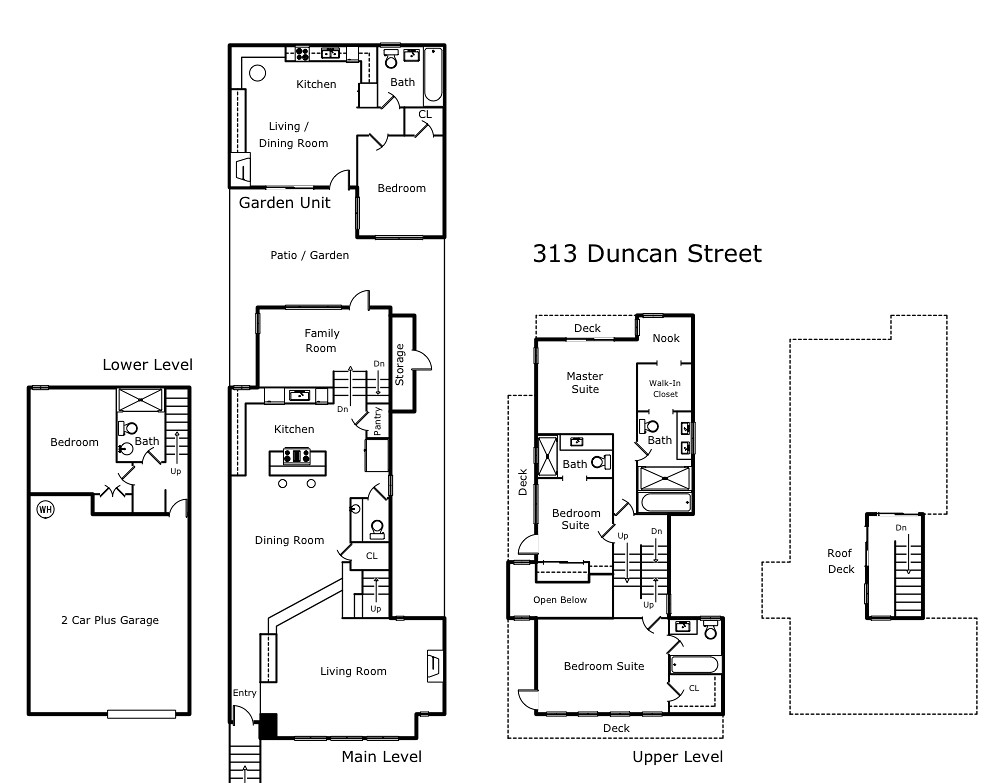Detailed Floor Plan of 313 Duncan Street

This image showcases a meticulously drawn black and white floor plan of a four-level house labeled "313 Duncan Street." The floor plan is divided into four distinct sections, each representing a different level of the house.

1. **Lower Level (Leftmost Drawing):**
   - **Bedroom:** Featuring ample space, suitable for guests or as a quiet retreat.
   - **Bathroom:** Adjacent to the bedroom, equipped with modern fixtures.
   - **Stairs:** Providing access to the main level.
   - **Garage:** Spacious enough to accommodate two cars, plus additional storage.

2. **Main Level (Second Drawing from the Left):**
   - **Kitchen:** Located at the top, designed for convenience with modern appliances.
   - **Living Area:** A comfortable space for relaxation and entertainment, adjacent to the kitchen.
   - **Bathroom:** Conveniently placed for guest and family use.
   - **Bedroom:** A cozy sleeping area, providing privacy and comfort.
   - **Patio Garden:** Below the living area, a small, yet charming outdoor space.
   - **Family Room:** Located below the patio garden, perfect for family gatherings.
   - **Dining Room:** Adjacent to the family room, designed for formal meals.
   - **Living Room:** Positioned below the dining room, a larger space for socializing and relaxation.

3. **Upper Level (Third Drawing from the Left):**
   - **Deck:** An outdoor area at the top, ideal for leisure and enjoying views.
   - **Master Suite:** Featuring a spacious bedroom, likely including an en-suite bathroom.
   - **Bathroom:** Located near the master suite for added convenience.
   - **Second Bedroom Suite:** Positioned at the bottom, another large bedroom perhaps with its own bathroom.

4. **Roof Level (Rightmost Drawing):**
   - **Roof Deck:** A vast, open deck area perfect for outdoor activities and entertaining, accessed via a set of stairs from the upper level.

This comprehensive floor plan provides a detailed and clear representation of the spatial organization and layout of the house at 313 Duncan Street, facilitating an easy understanding of each level's function and features.